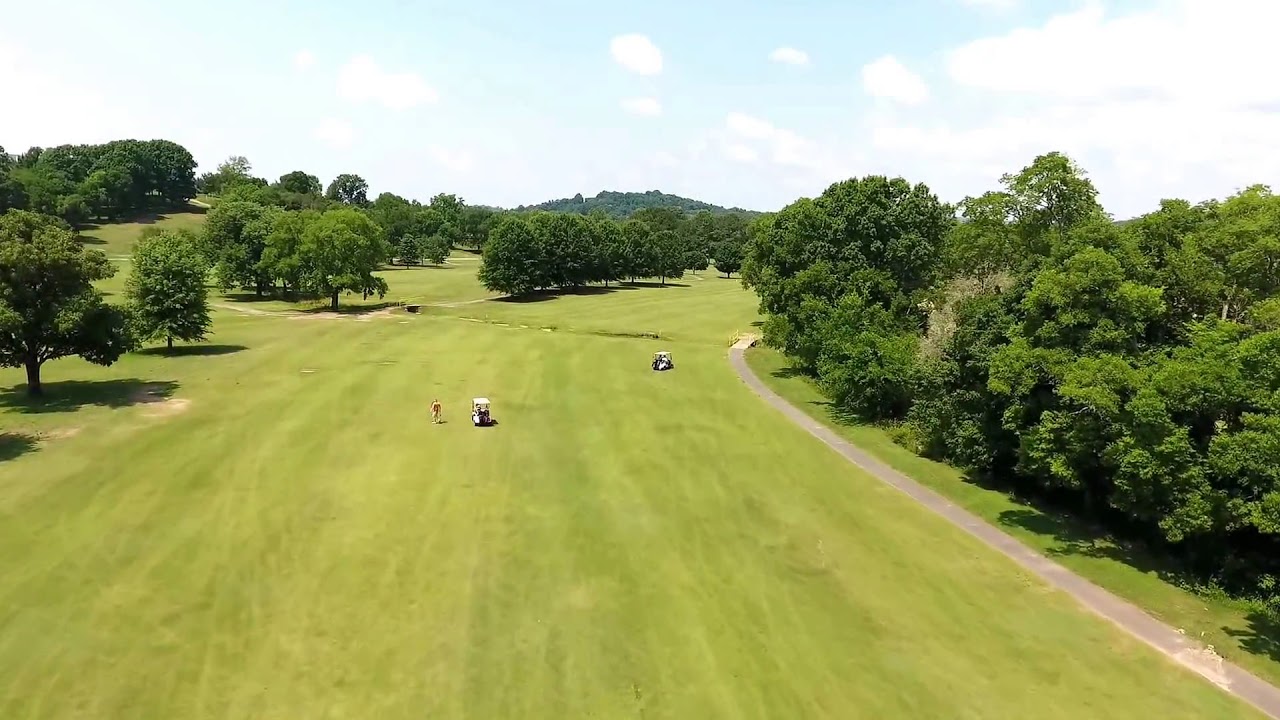This vibrant photograph captures an expansive view of a golf course from an elevated perspective, resembling a tree-top viewpoint. Dominating the middle of the image is the lush, manicured greenery of the golfing green, with a small cement sidewalk running adjacent to it. The scene is framed by clusters of very green trees on both sides, with a particular density of trees to the right of the sidewalk. In the center, two golf carts can be seen: one nearer to the middle with a person walking beside it, and another farther in the distance. The landscape at the back curves gently to the right, with the foliage following suit. Overhead, a mostly blue sky is lightly accented by scattered white clouds, indicating a clear, sunny day. The image depicts the various colors vividly, highlighting the green hues of the vegetation, the beige and brown elements potentially from the earth or golf equipment, gray for the sidewalk, and multiple shades of blue and white in the sky.